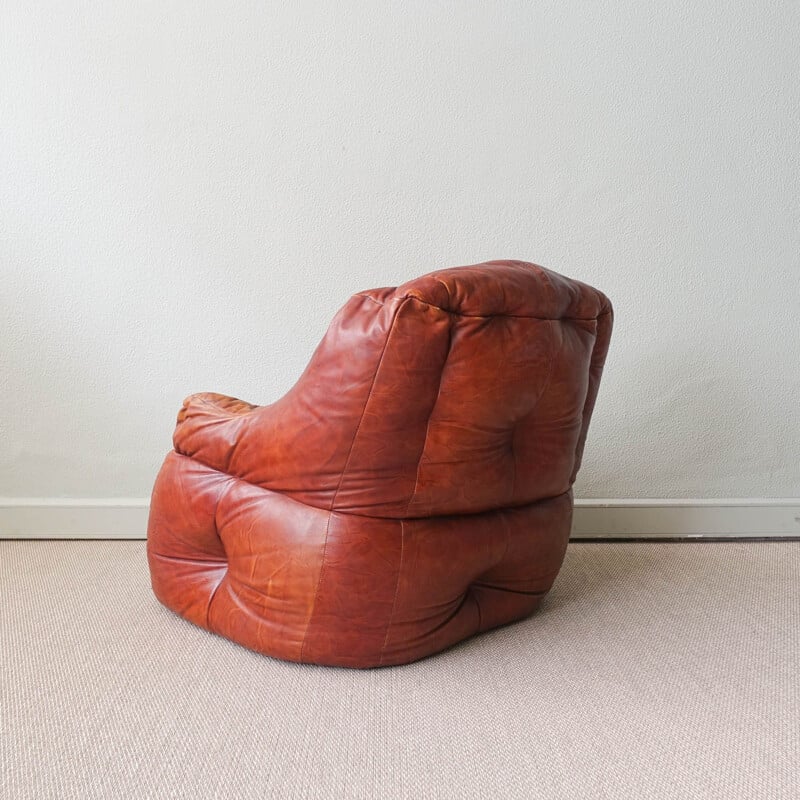The photograph showcases a close-up of the back and left side of a unique brown leather beanbag-style chair. Unlike conventional beanbag chairs, this one is shaped more like a hybrid between a beanbag and a lounge chair, featuring a structured back and armrests that resemble a sofa top. The leather appears well-worn and has a reddish-brown, almost rust-like hue, indicative of a vintage aesthetic from the 70s. Positioned against a plain, textured white wall, the room is minimally decorated, with only a white molding at the base. The chair rests on thin, high-traffic area carpeting that has a very light beige or wheat color, possibly with a chevron pattern. The focus of the image is clearly on the chair, highlighting its high-quality material and comfortable, albeit rumpled, appearance. The simple and uncluttered setting emphasizes the chair's unique design and rustic charm.